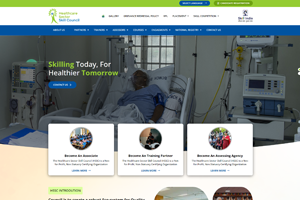The image captures a webpage from a health-related website, though the text is almost unreadable due to its blurry and tiny appearance. The interface features a green header bar at the top, containing two prominent buttons—one blue and one green. Beneath this header bar is the website's logo, followed by a menu with five main topics. Below the menu, a blue bar lists eight categories.

The main content area of the homepage displays a photograph of a person with dark skin lying in an elevated hospital bed, wearing a gown. The room is dimly lit. Superimposed on the image is a motivational sentence: “Skilling Today, For Healthier Tomorrow.” The words "Skilling" and "Tomorrow" are in green text, while "Today" and "For Healthier" are in white. Just below this text overlay is a prominent blue button.

Additionally, beneath the image, there are three equally-sized square options, indicating further selections or actions available on the site.